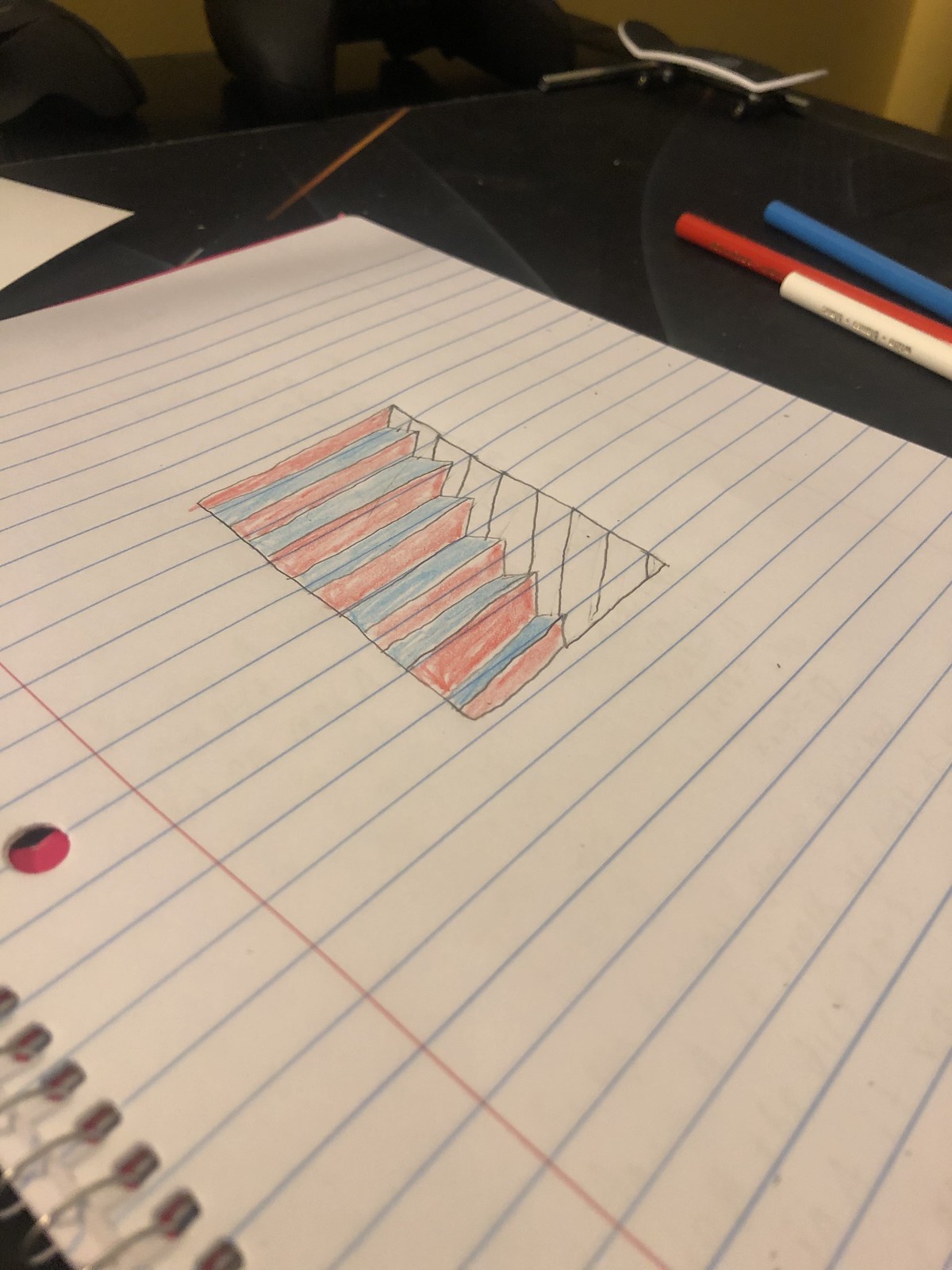This image features a rectangular portrait of a sheet of lined notebook paper, still attached to its spiral binding. The paper is tilted at a precise 45-degree angle, with the upper right corner nearly vertical. The sheet's edges are truncated, revealing only a portion of both the top and the right side, while the bottom left corner showcases the spiral binding and one of the three punched holes. 

The paper itself is standard with blue horizontal lines and a single red vertical line marking the margin on the left. Positioned towards the upper middle section of the paper, there is a hand-drawn depiction of a descending staircase. This drawing occupies about one-third of the paper’s width, delineated from the red margin to the right edge. The illustration is executed in pencil, with the steps colored using blue for the tops and red for the risers, giving a clear sense of depth. Six steps are visible, enhanced by vertical pencil lines on the right side, simulating a wall and further accentuating the staircase's descending nature.

The notebook paper rests on what appears to be a black table. In the top right corner of the image, three writing implements are partially visible. These include a medium blue pen or pencil at the top, a red one in the middle, and a white one at the bottom. Their tips are out of the frame, suggesting they might have been used for the drawing on the notebook paper.